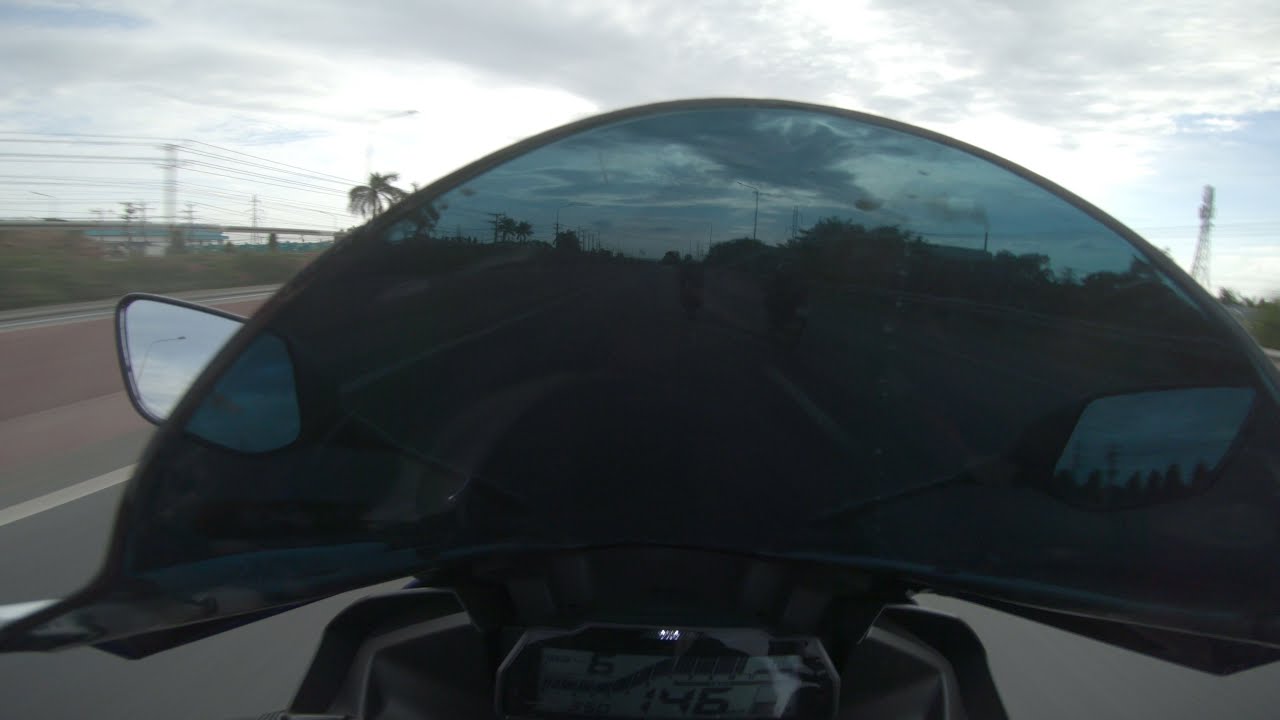The image captures a wide rectangular photograph taken from the perspective of someone sitting on a black motorcycle. The front of the motorcycle is at the bottom of the image, featuring a semi-circular, tinted blue windshield through which the road ahead is visible, including the side mirrors on both the left and right. Below this windshield, a display screen showing the number 146 is visible, likely indicating the bike's speed. Surrounding the highway, there are other vehicles, including other motorcyclists. The highway itself is gray with white lines, bordered by green grassy areas dotted with trees and palm trees. On the right side, there is a tall cell phone tower, while the left side has more highway sections, including a bridge, and additional electrical towers and wires. The sky above is a mix of light blue and densely packed white and blue-gray clouds.